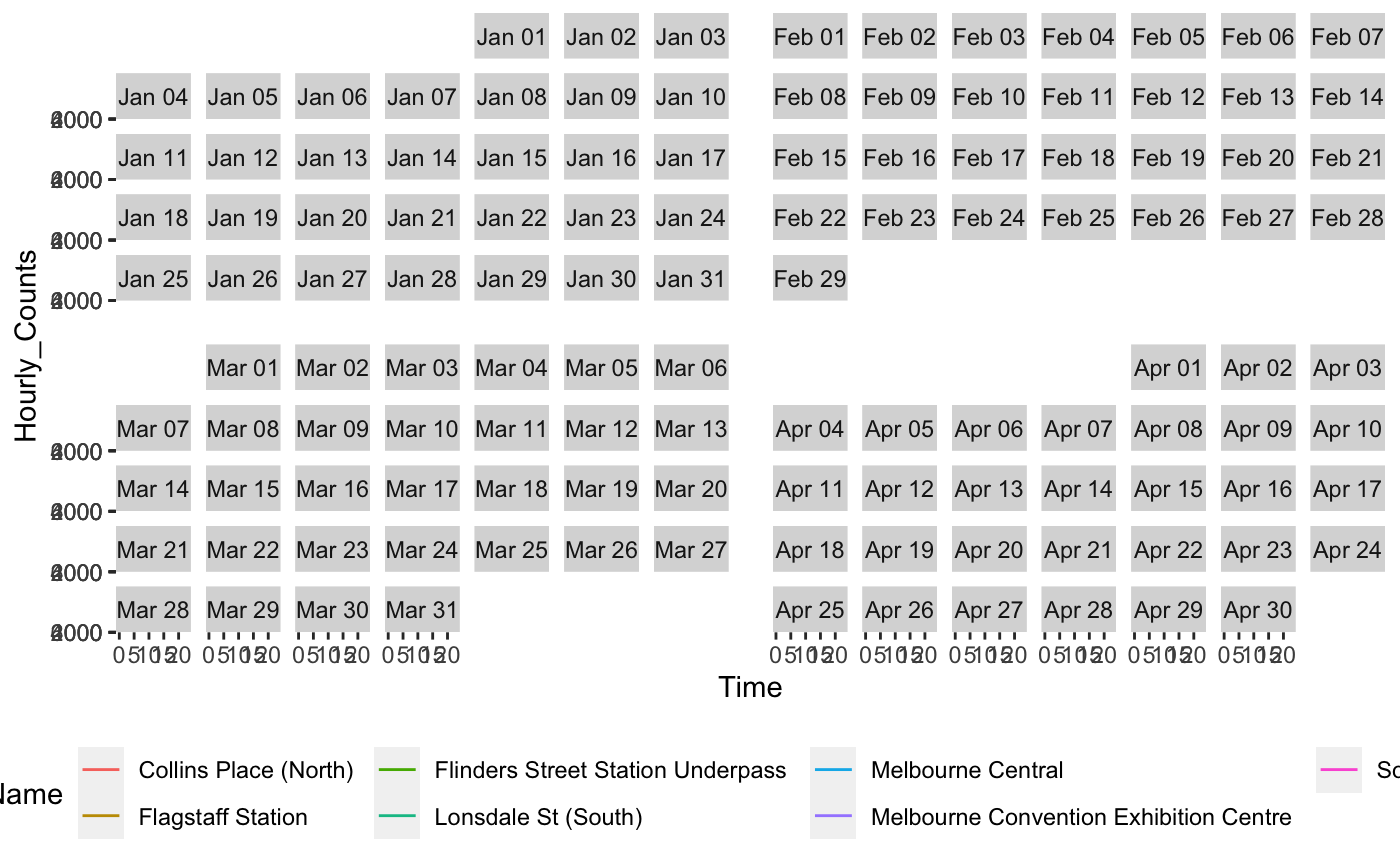The image is a composite calendar spanning four months—January, February, March, and April. The layout is split with January and February positioned at the top and March and April side-by-side at the bottom. Along the left-hand edge of the screenshot, the term "Hourly Counts" is displayed vertically, indicating some form of hourly measurement. Each date within the calendar is enclosed in its own rectangular gray square, offering a clear, organized visual of the months.

At the bottom-center of the page, the word "Time" is prominently noted. Just above this, there are three vertical rectangles, each extending horizontally across the bottom of the screen. These rectangles are sectioned by two internal lines apiece. The first rectangle on the left features orange lines, the middle has green lines, and the rightmost rectangle is marked by blue lines. Adjacent to these colored sections, text labels provide specific locations: Collins Place North, Flagstaff Station, Flinders Street Station Underpass, Lonsdale Street South, Melbourne Central, and Melbourne Convention and Exhibition Centre.

The detailed composition and labeling suggest this calendar might be used for tracking or displaying hourly counts of specific events or activities occurring at these various Melbourne locations within the first four months of the year.